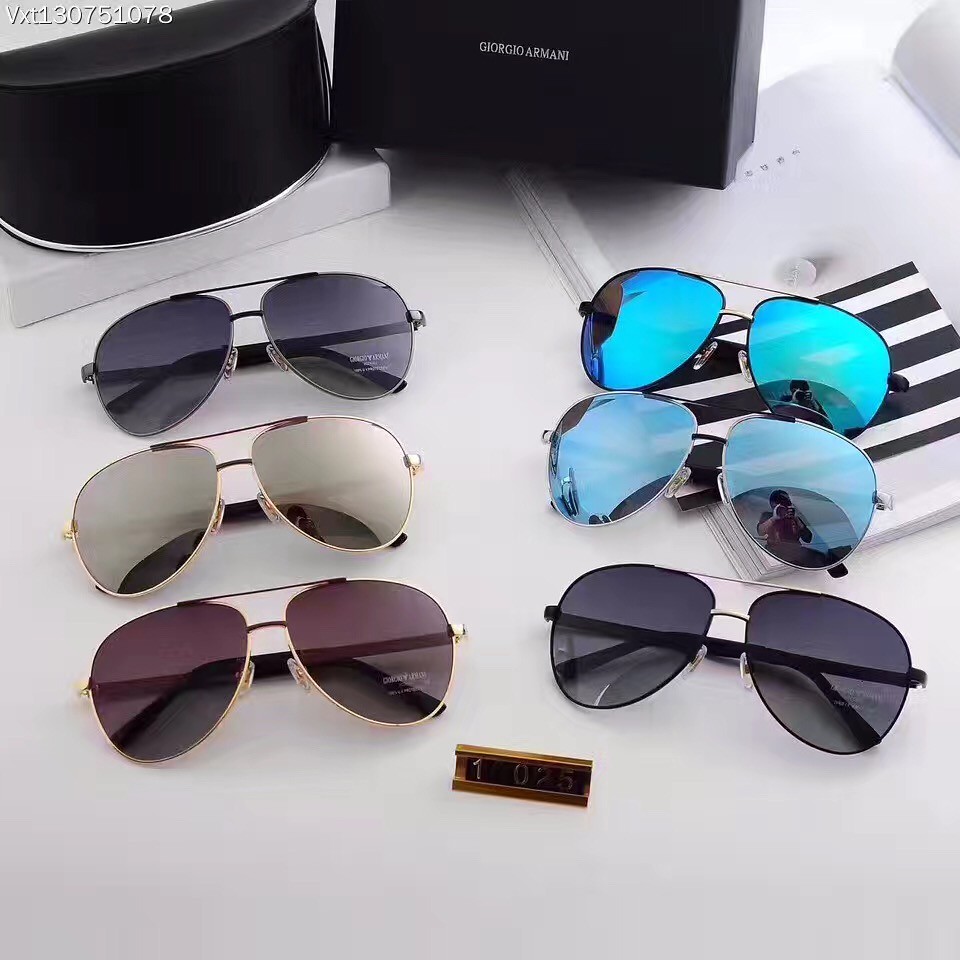The photograph features a meticulously arranged display of six pairs of designer sunglasses, positioned on a pristine white surface. Each pair of sunglasses, varied in tint and style, demonstrates a range of colors including light shades, bluish hues, dark red, silver, purple, deep amber, and reflective bluish-green. The top left pair of sunglasses is marked with an unclear writing on one of its lenses. The arrangement of the sunglasses shows them aligned in two rows or columns, with two pairs resting atop an open book.

In the background, two black cases add to the elegant setting. The right case, square in shape, features the brand name "Giorgio Armani" inscribed in white letters. Contrastingly, the case on the left has a half-circle shape. Above the display, the alphanumeric sequence "VXT130751078" is written in white. Reflections of the person holding the camera are discernible in several of the sunglass lenses, adding a subtle human element to the composition. At the bottom of the display sits a small wooden placard bearing the number "1025," further complementing the aesthetic arrangement of the scene. This detailed setup suggests an advertisement for high-end designer sunglasses.